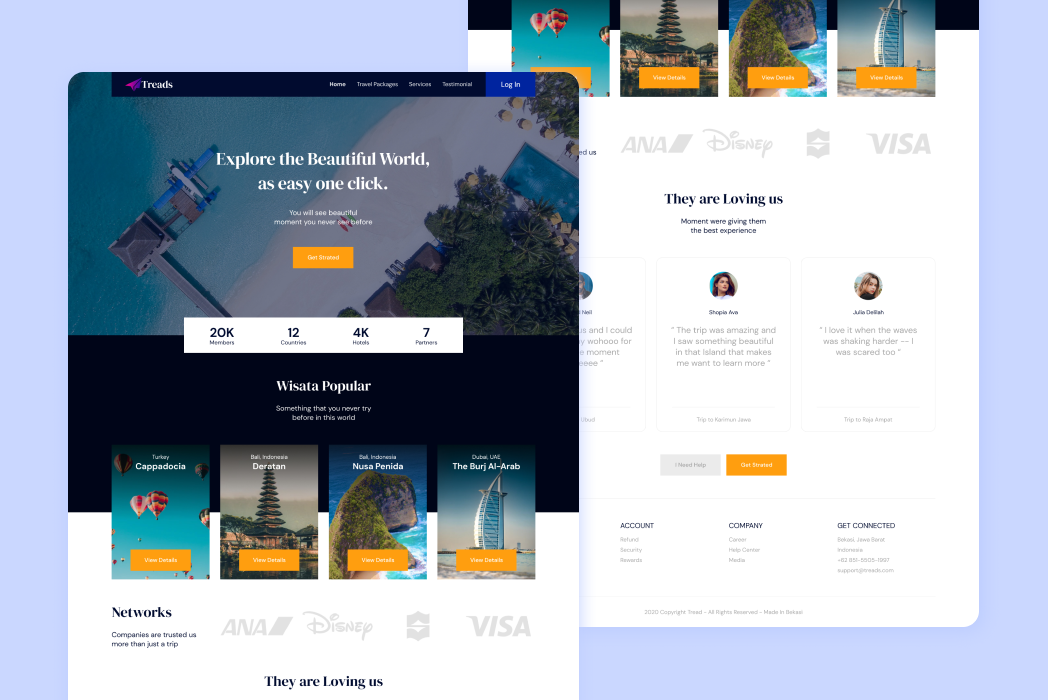**Image Description:**

The image is a detailed screenshot from a computer with a light blue background. It primarily focuses on what appears to be two overlapping A4 sheets, positioned at different angles. The left sheet fully aligns with the bottom border of the rectangular background, while the right sheet is slightly cut off at the top, showing a portion of the blue background at the bottom.

### Top Section:
- **Header Background**: Black area at the top.
- **Logo and Company Name**: Featured prominently.
- **Categories**: Divided into four white sub-categories.
- **Login Button**: Blue with white text "LOGIN".

### Main Content:
- **Background Image**: Shows a sky with clouds, greenery, various buildings, and a tower.
- **Slogan**: Large white text "EXPLORE THE BEAUTIFUL WORLD" and below it "As easy as one click."
- **Small Text**: Two lines of unreadable white text with a logo of three purple dots.
- **Action Button**: An orange rectangle with white text.
- **Statistics Section**: White background rectangle featuring dark letters and numbers:
  - "20k" with details below.
  - "12" with details below.
  - "4K" with details below.
  - "7" with details below.

### Middle Section:
- **Category Label**: Black area stating "POPULAR".
- **Images and Labels**: Four labeled images with orange rectangular boxes at the bottom:
  - Hot air balloons against a blue sky.
  - A tall pointed structure.
  - An ocean scene with rocks and grass.
  - A pointed silver and blue object.
- **Additional Text**: Black text "NETWORKS" with additional notes, including:
  - Light gray "ANA" with a slanted gray box.
  - "Disney" in cursive to the right.
  - Two gray roofs, one below the other.
  - "VISA" in gray, all caps.
  - "They are loving us" in black.

### Testimonials Section:
- **Circular Photos**: Three photos with light gray borders, names and testimonials underneath.
- **Boxes**: Adjacent gray and orange boxes with text.

### Bottom Section:
- **Account and Connection Options**: Labeled "ACCOUNT" in caps, "Company", and "Get Connected".
- **Categories**: Three categories under the first two options, four under the last.
- **Footer Text**: Light gray text at the bottom. 

Overall, the screenshot depicts a user-friendly and engaging interface with a variety of visual and textual elements that guide the user through exploring content, statistical information, promotional features, and user testimonials.